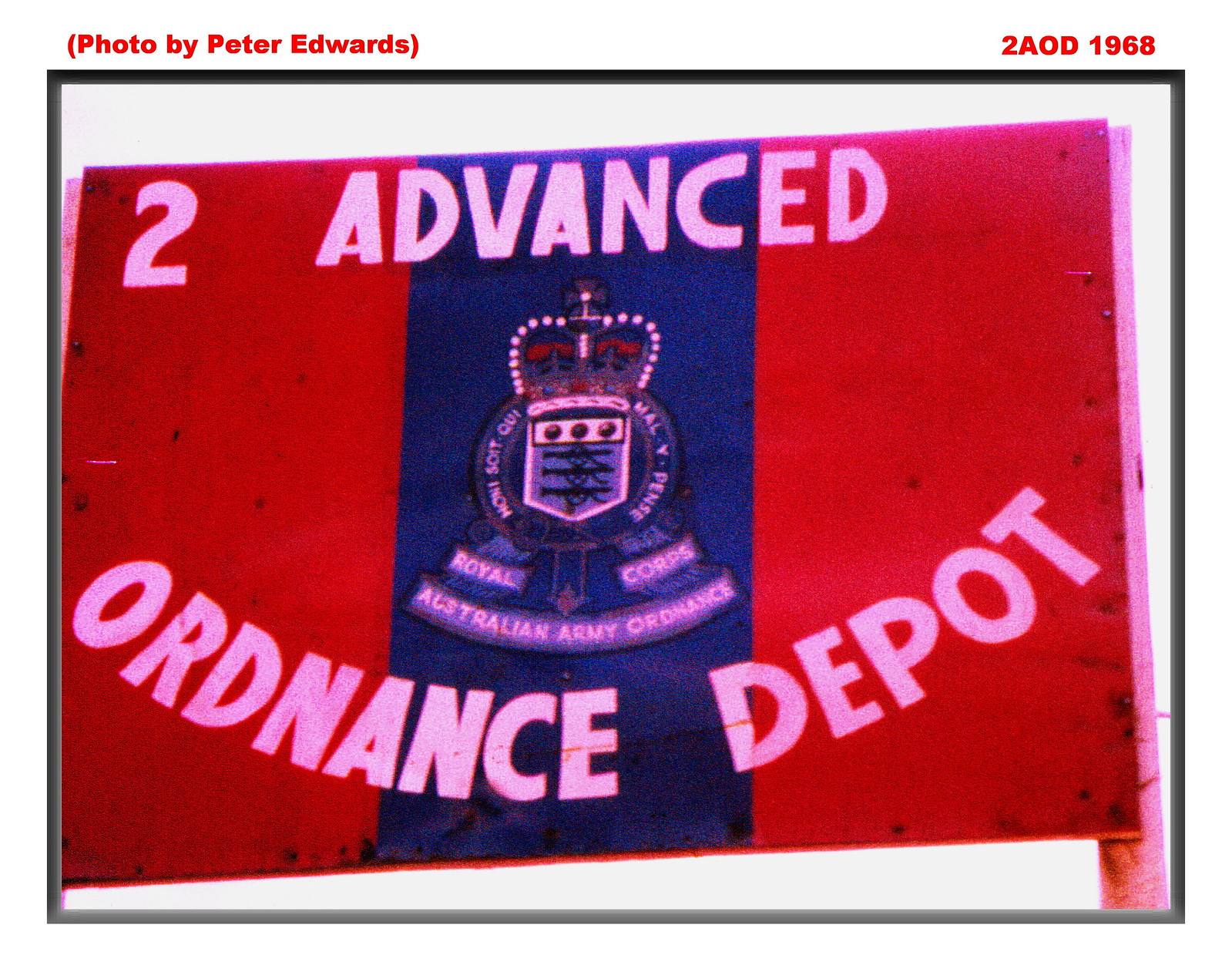This image is a possibly computer-generated or digitally created picture of a flag, bordered by a black frame and set against a white background. At the very top, in red letters and in parentheses, it is captioned "photo by Peter Edwards." In the top right corner, also in red letters, it reads "2AOD 1968."

The flag itself is divided vertically into three equal sections: the left and right sections are bright red, and the middle section is blue. The central blue section features a crest bearing the image of a crown, indicative of the Royal Corps of Australian Army Ordnance. Accompanying the crest are inscriptions including symbols like guns and crown jewels, though they appear a bit unclear.

Spanning across the top of the flag in bold white text, it reads "2Advanced." At the bottom, in white text with a slight curve resembling a smile, it states "Ordnance Depot."